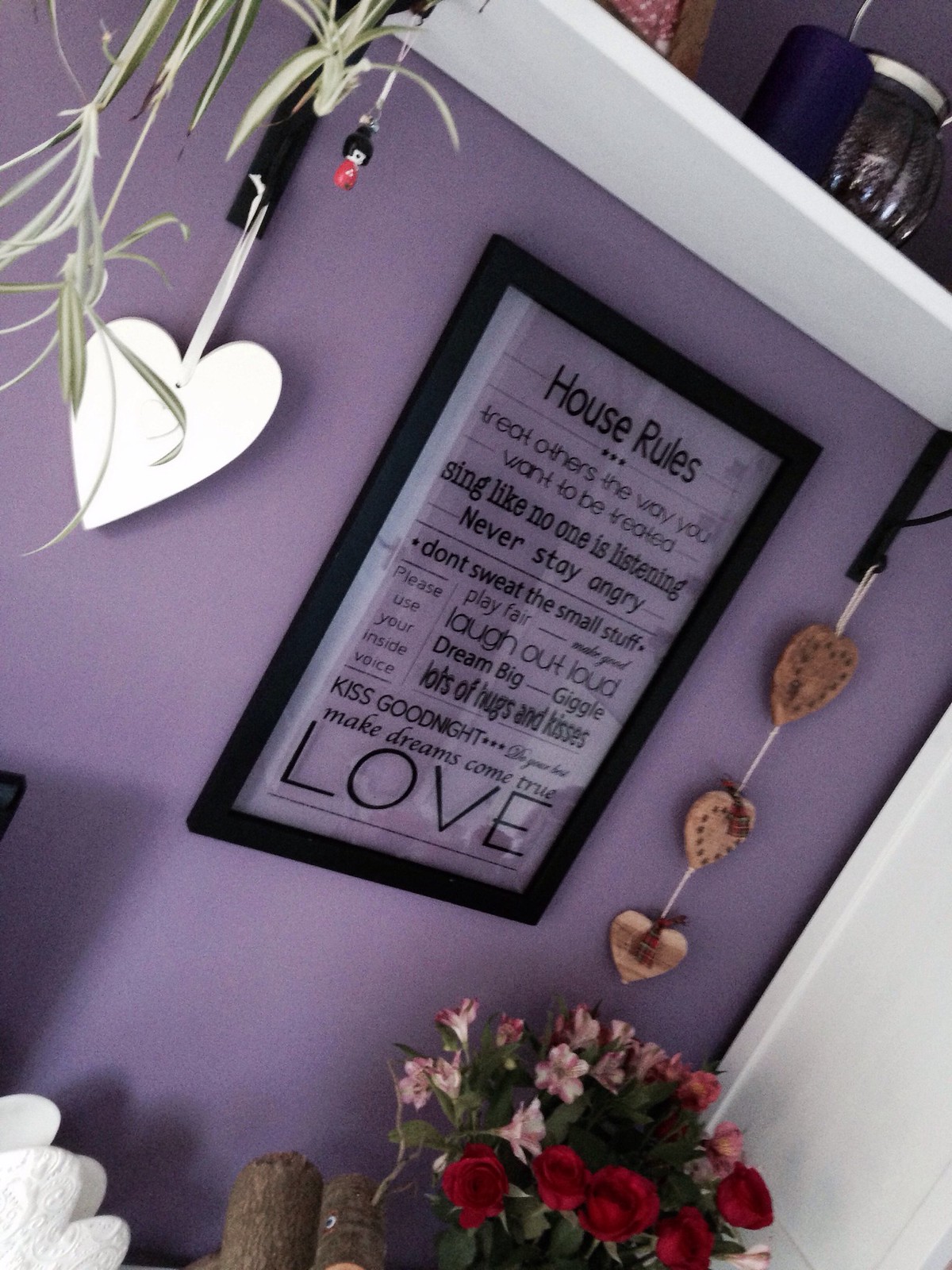This image depicts a cozy, off-center scene with a beautifully detailed lavender-colored wall as the backdrop. A white shelf adorned with a vase and a cup is the focal point, and from its brackets, intricately carved wooden heart decorations dangle elegantly. To the left of the shelf, dangling foliage adds a touch of greenery. Dominating the lower right corner, a bouquet of vibrant roses and assorted flowers adds a burst of color. Mounted on the wall beneath the shelf is a black-framed sign with the text "House Rules: Treat others the way you want to be treated. Sing like no one is listening. Never stay angry. Don't sweat the small stuff. Please use your inside voice. Play fair. Laugh out loud. Dream big. Giggle. Lots of hugs and kisses. Kiss goodnight. Make dreams come true. Love." The image, slightly tilted to the right, creates a charming, whimsical aesthetic.